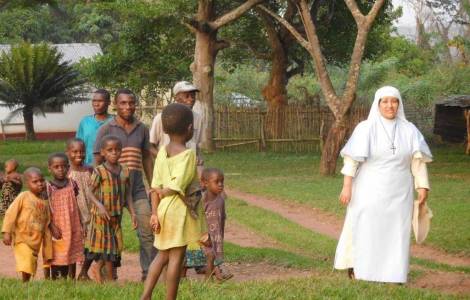This photograph captures a serene outdoor scene bathed in clear, sunny daylight. A lighter-skinned woman dressed in full nun's attire, adorned with a crucifix and clutching a beige object, stands prominently on the right. Her head is covered and she wears a white gown that envelops her completely. Across from her on the left, a diverse group of children and a few adults, all with brown skin, stand facing her. The children and adults are likely of African heritage. The scene unfolds on a well-maintained grassy area, intersected by a dirt path. In the background, a wooden fence encloses the area, and large trees, including a distinctive short, wide date palm, stand tall against a backdrop of woods and a house. This setting, possibly suggesting a missionary or educational context, exudes a peaceful, communal atmosphere.